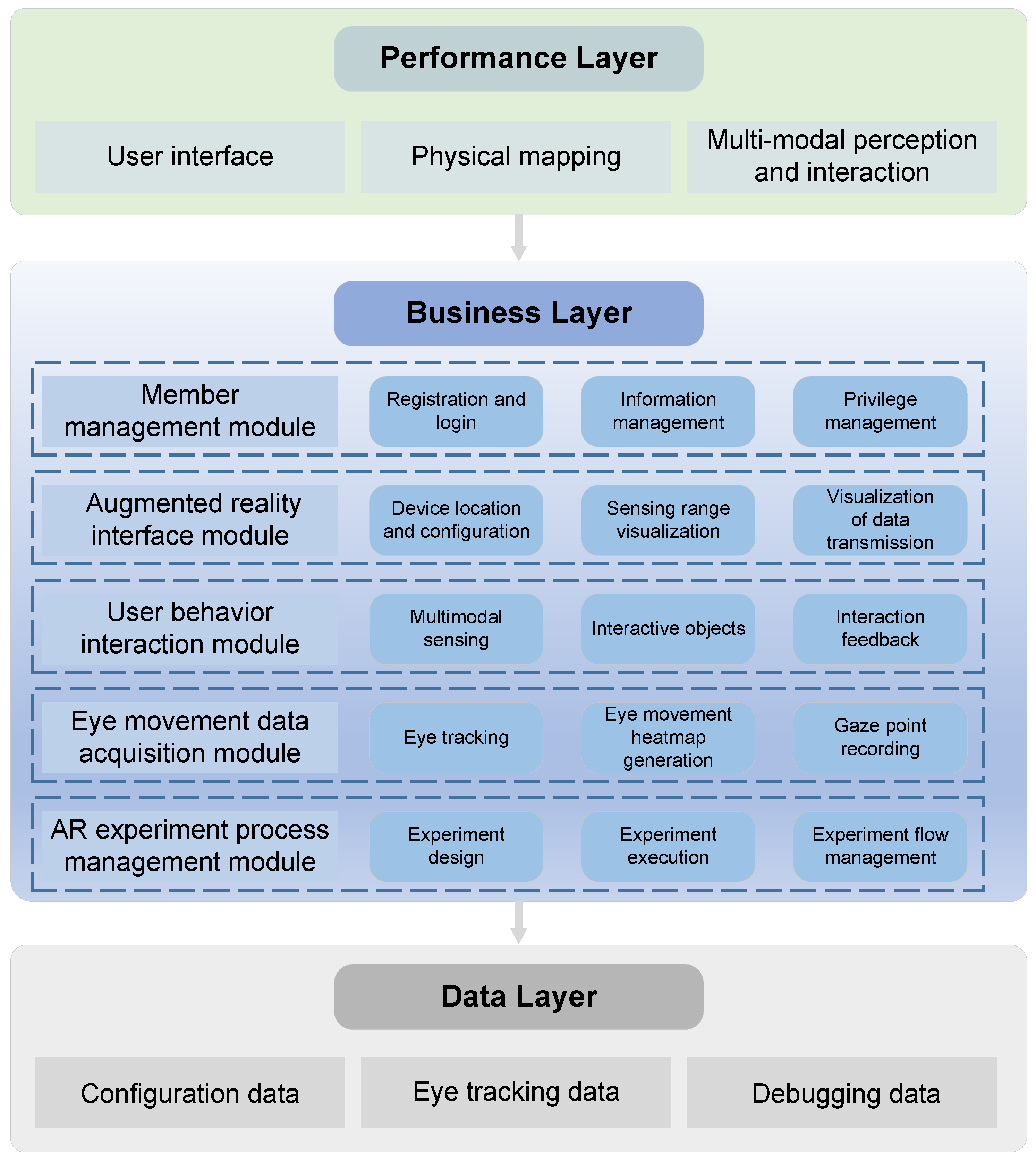The image is a vertically rectangular, multi-layered diagram outlining three distinct layers: the performance layer, the business layer, and the data layer. Each layer is marked in different colors- the performance layer in light green, the business layer in purple, and the data layer in gray- with black text throughout.

At the very top lies the performance layer, a horizontal, light green rectangle featuring smaller bluish-green bubbles. Inside, from left to right, are labeled segments reading: "user interface," "physical mapping," and "multimodal perception and interaction." Below this is a gray arrow pointing downward towards the business layer.

The business layer, the largest section, includes multiple fields organized in rows. These fields include:
- Member management module
- Registration and login
- Information management
- Privilege management
- Augmented reality interface module
- Device location and configuration
- Sensing range visualization
- Visualization of data transmission
- User behavior interaction module
- Multimodal sensing
- Interactive objects
- Interaction feedback
- Eye movement data acquisition model, encompassing:
  - Eye tracking
  - Eye movement heat map generation
  - Gaze point recording
- AR experiment process management module, encompassing:
  - Experiment design
  - Experiment execution
  - Experiment flow management

The final section, delineated as the data layer, lists key areas such as configuration data, eye tracking data, and debugging data.

This diagram visually organizes the elements and modules of a multimodal business interface, ensuring clarity with distinct layers and color-coded sections.